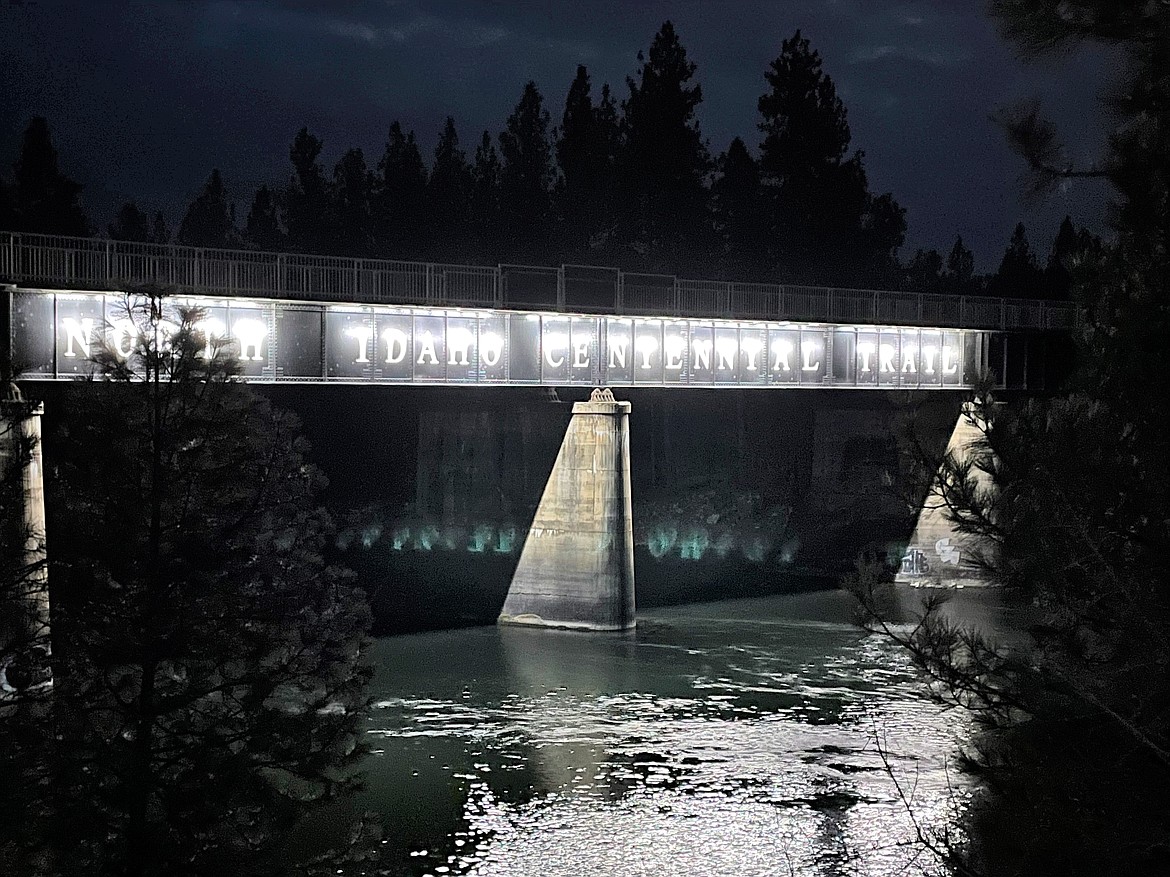This nighttime photograph captures an evocatively lit, repurposed railroad bridge, now serving as part of the North Idaho Centennial Trail. The bridge, which retains its historical metal framework, spans a serene river, its structure supported by sturdy cement pillars emerging from the water below. Above, protective metal railings line the bridge, ensuring the safety of individuals using it as a pedestrian walkway. The surrounding darkness of the night is gently illuminated by the lights on the bridge, casting a tranquil glow on the scene. Trees frame the image on both sides, shrouded in shadows, while additional trees are visible in the background, standing sentinel behind the bridge. The still water underneath reflects the faint light, adding to the serene and timeless atmosphere of this picturesque scene.